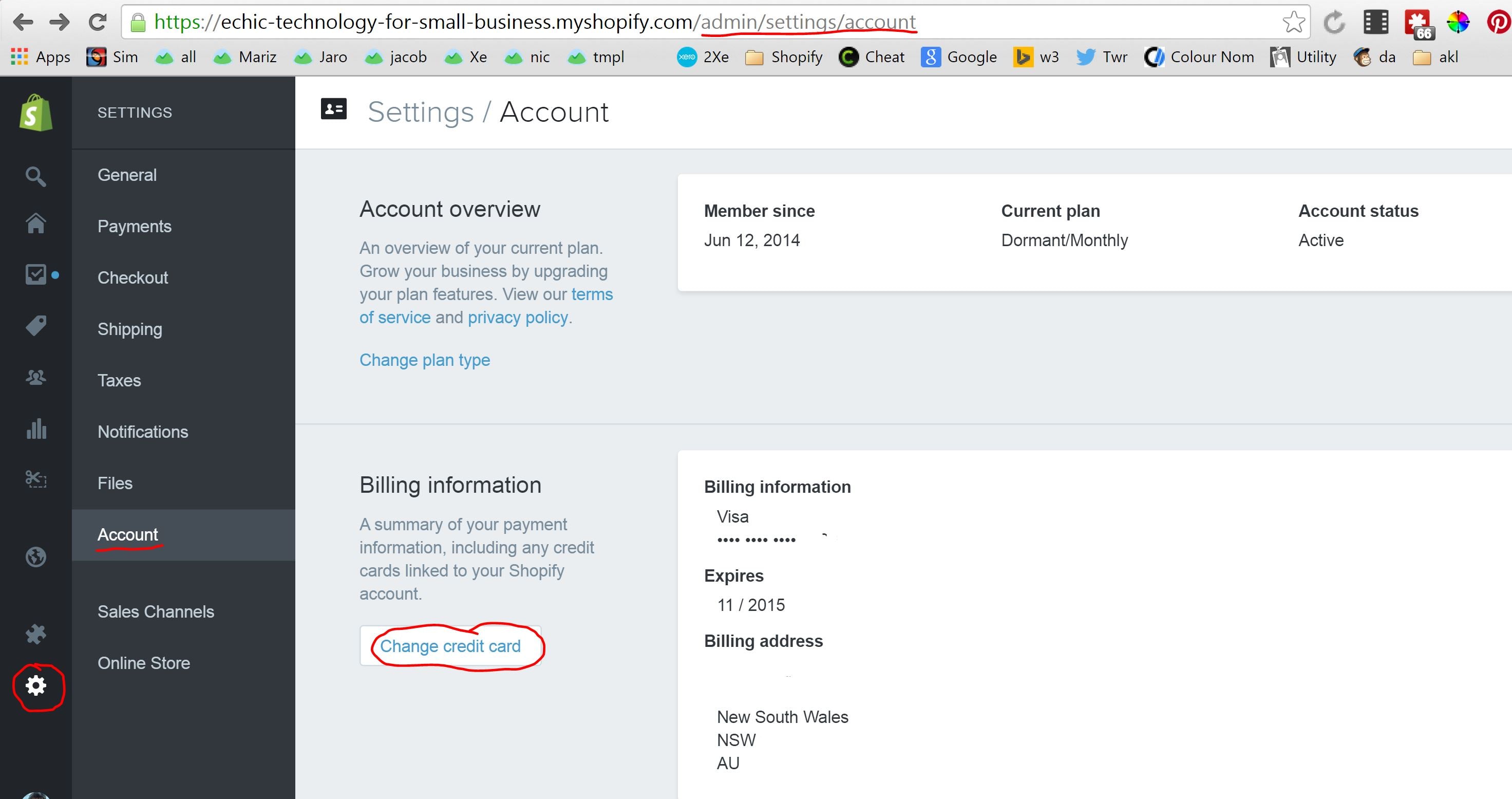This image depicts the admin settings page of an individual's Shopify site. The URL bar is highlighted with a red underline focusing on the segment "admin/settings/account," indicating that this specific section is being accessed. The settings cogwheel icon is circled in red for emphasis, guiding the user to this particular area. Beneath the billing information, there's a noticeably crude red circle drawn around the credit card details section, pointing out where to update or amend payment information. The Shopify store, named "E-Chic Technology for Small Business," has been active since June 12, 2014. This detailed and annotated screenshot is aimed at helping the user navigate their Shopify account settings, specifically to update billing information.